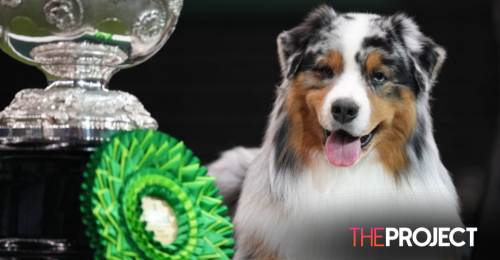The image, titled "THE PROJECT" as indicated by the red and white uppercase text in the bottom right corner, depicts a striking scene with a predominantly black background. Central to the composition is a young dog, likely an Australian Shepherd or Collie mix, gazing directly at the viewer with its pink tongue playfully out. The dog's fur is a beautiful blend of white, chestnut brown, and black, with a distinctive white streak running from its chest up between its eyes. Its ears, mostly black with some white, contribute to its endearing appearance.

Beside the dog, on its left, is a prominent circular green ribbon with a central white circle, suggesting an award. In the top left quadrant of the image, partially obscured, is the bottom half of a silver trophy, hinting at an accomplished feat. The overall aesthetic of the poster is somewhat nostalgic, evoking a retro, possibly 80s feel due to its design and color scheme. The dog's poised stance beside these prizes suggests it has won or is being celebrated for a significant achievement.